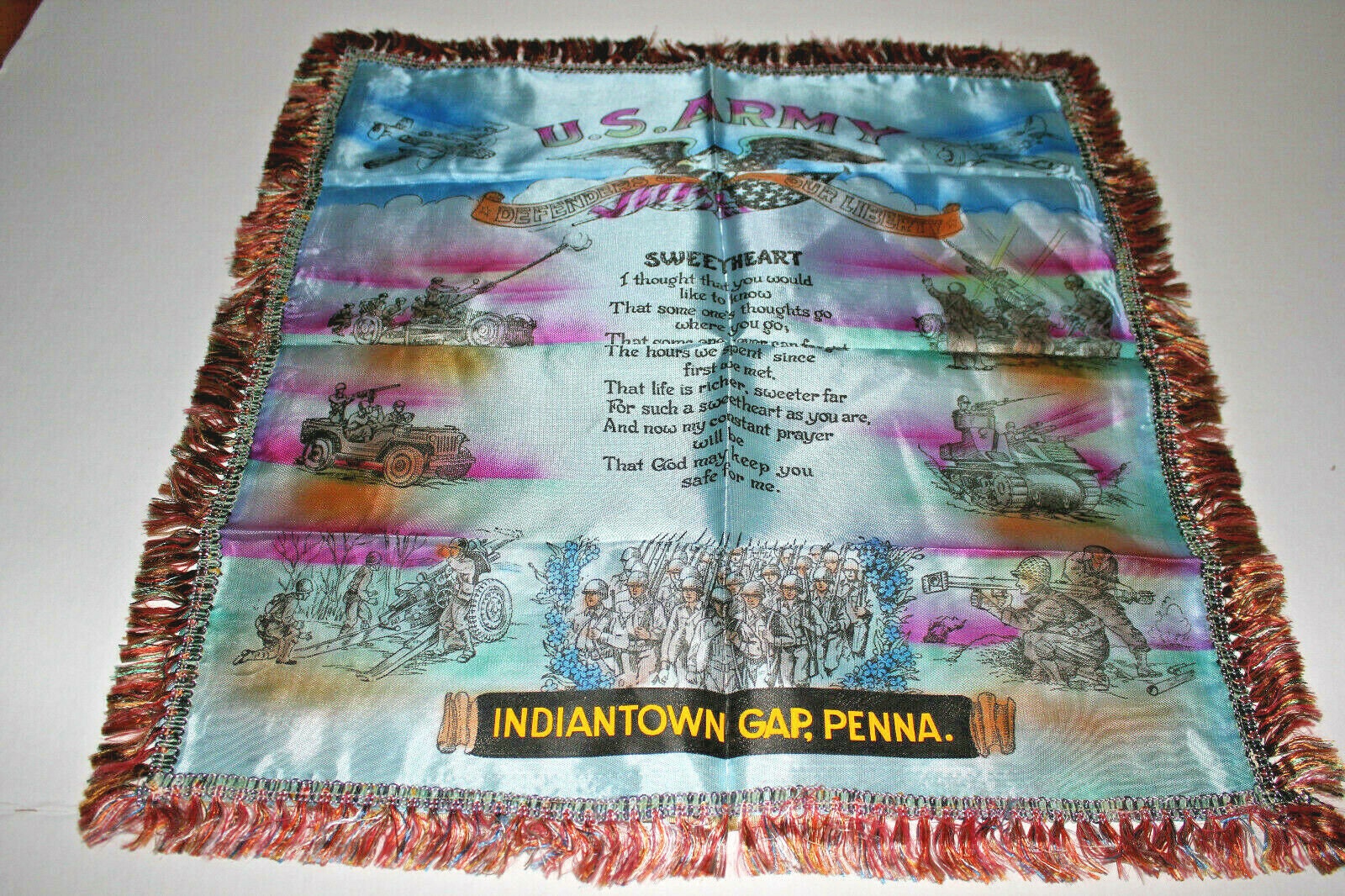This detailed and colorful image depicts a U.S. Army tapestry, possibly a poster, blanket, or rug, featuring hand-drawn artwork that is primarily framed in red fringe with accents of blue, orange, yellow, pink, and silver. The rectangular tapestry appears to be lying flat on a white table or hanging on a white wall, creating some ambiguity about its orientation. Central to the tapestry is a poem titled "Sweetheart," written in black text with some folds obscuring parts of the poem. The top section features a pair of old warplanes, while the left side showcases an army jeep with a man standing at the back holding a gun and another person driving. Surrounding the central poem are various army vehicles, including trailers equipped with gun turrets. The right side of the tapestry shows soldiers manning another gun turret, below which is an army tank, followed by a soldier with a bazooka at the bottom right. In the bottom middle, a company of soldiers is seen marching. The tapestry bears the inscription "Indian Town Gap Penna," referring to Indiantown Gap, Pennsylvania, using an older abbreviation for the state. Despite being an army-themed item, it is unusually bright and colorful with stylistic choices that are not typically associated with U.S. military artifacts.